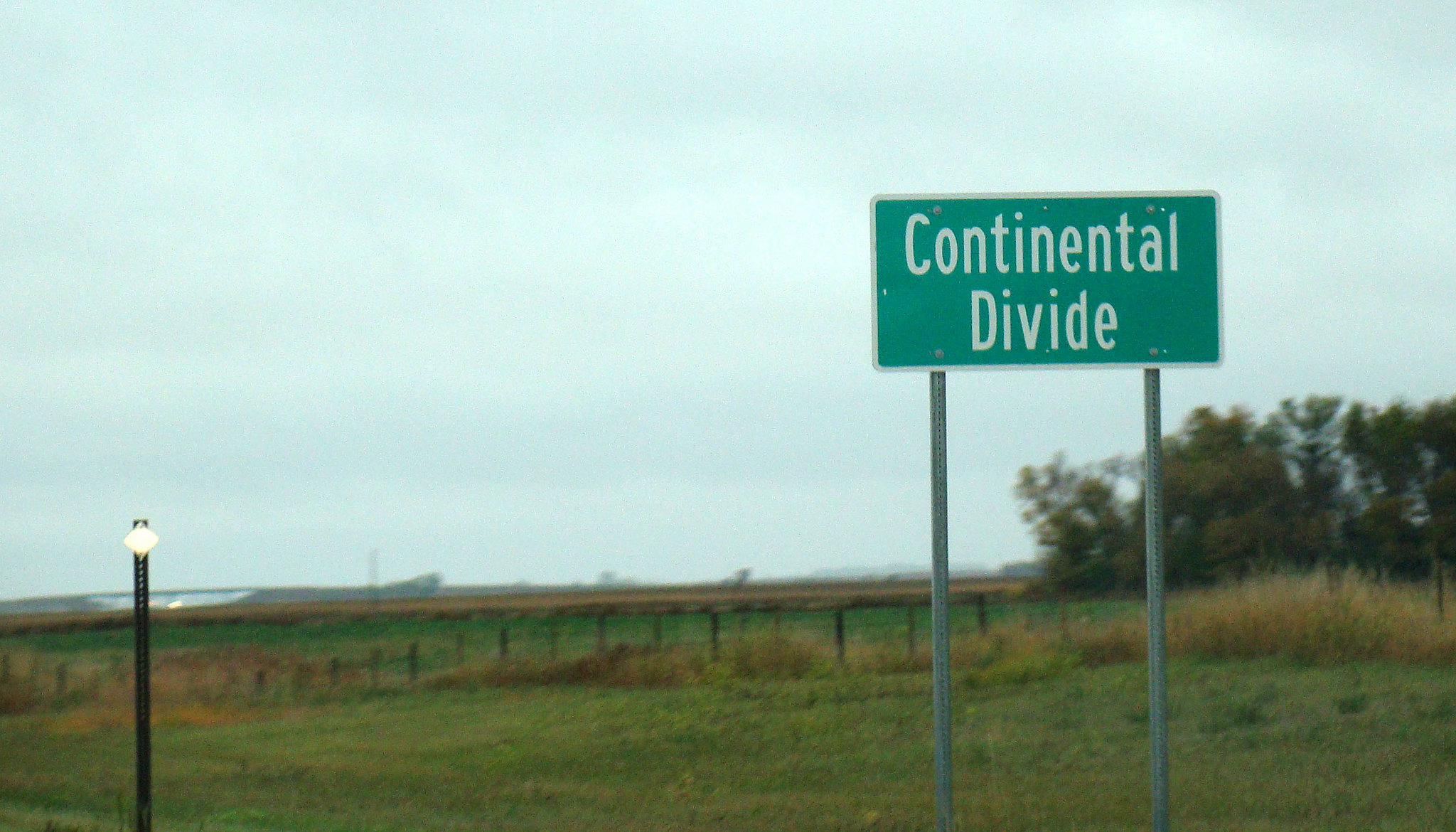The photograph captures an expansive countryside field under a grey, cloudy sky that casts a subdued light over the scene. At the forefront on the right-hand side, a sign prominently stands on two slender metal posts, colored green with white letters reading "Continental Divide." The image has a slight grainy texture and blur, giving it a somewhat vintage feel. To the left, the field teems with tall, overgrown grass, some of it dry, indicating a lack of recent mowing. A fence bisects the field midway, beyond which more open, green terrain stretches out. In the background, possibly an overpass or freeway appears faintly, with distant lights of oncoming vehicles. Additionally, a black pole with a diamond-shaped light is visible on the left side, suggesting it might serve as a safety or navigation light. Scattered across the scene are several mid-sized trees, adding to the rustic charm of the landscape.